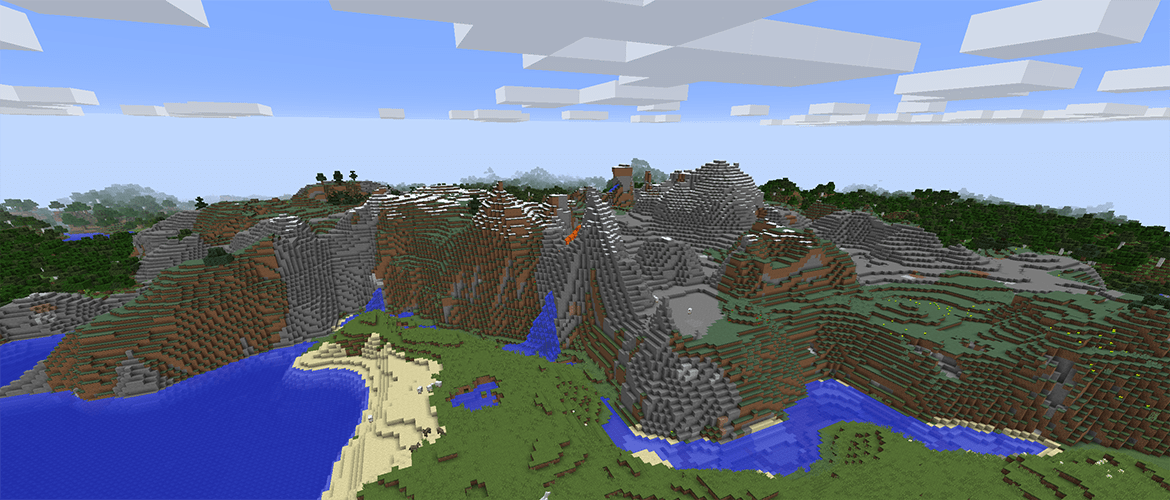This panoramic image captures a detailed, angled downward view of a Minecraft landscape from a high vantage point, almost at the level of the clouds which recede into the distance. The scene showcases a diverse terrain, featuring a series of rugged, gray-colored mountain ranges extending into brown and green terraced hills, capped with occasional trees and patches of vegetation. In the lower left, a large body of bright blue water is bordered by a lengthy stretch of white sandy coastline, with various smaller lakes, streams, or waterfalls cascading down the cliff faces. The sky is a patchwork of blue and dark clouds, adding depth to the expansive vista. The overall color palette includes grays, browns, whites, greens, and blues, creating a visually rich and varied landscape that highlights both the natural beauty and the blocky, unique aesthetic of the Minecraft world.